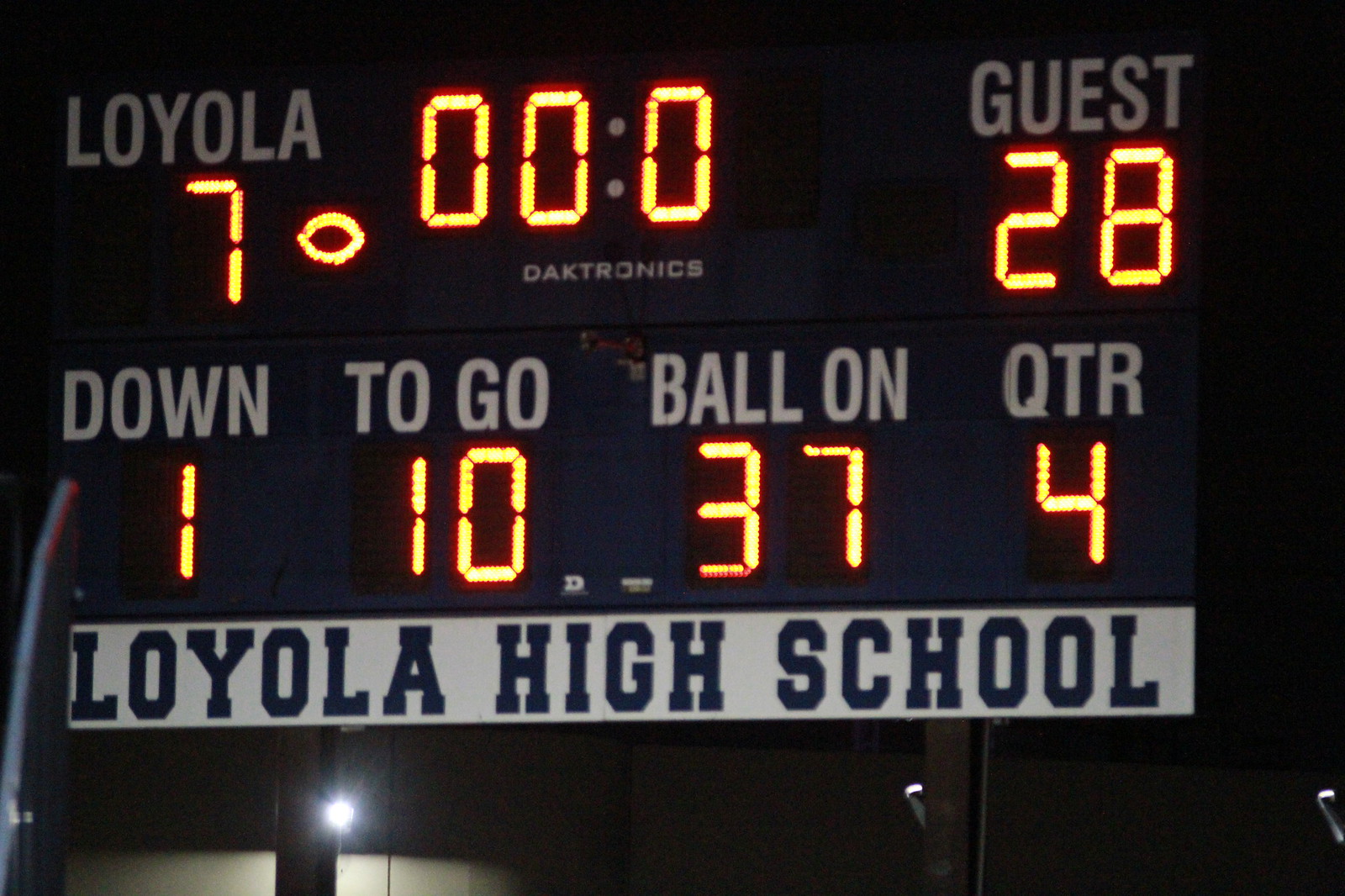This is a color photograph of an outdoor high school football scoreboard taken at night, featuring black background with orange LED lighting. At the top left of the scoreboard is the home team, Loyola, with a score of 7 points, indicated by an orange number with a small football icon next to it. On the top right, the score for the Guest team stands at 28 points. The time clock at the top center shows 00:00, and the name "Datatronics" appears beneath it. Below the scores, detailed game statistics are displayed: it is the first down with 10 yards to go, the ball is on the 37-yard line, and it is the fourth quarter. At the bottom of the scoreboard, a white banner with black lettering reads "Loyola High School." There is a small glimmer of background light in the lower left-hand corner, and the overall appearance of the scoreboard suggests it might be somewhat dated, with a possibly 1980s style.